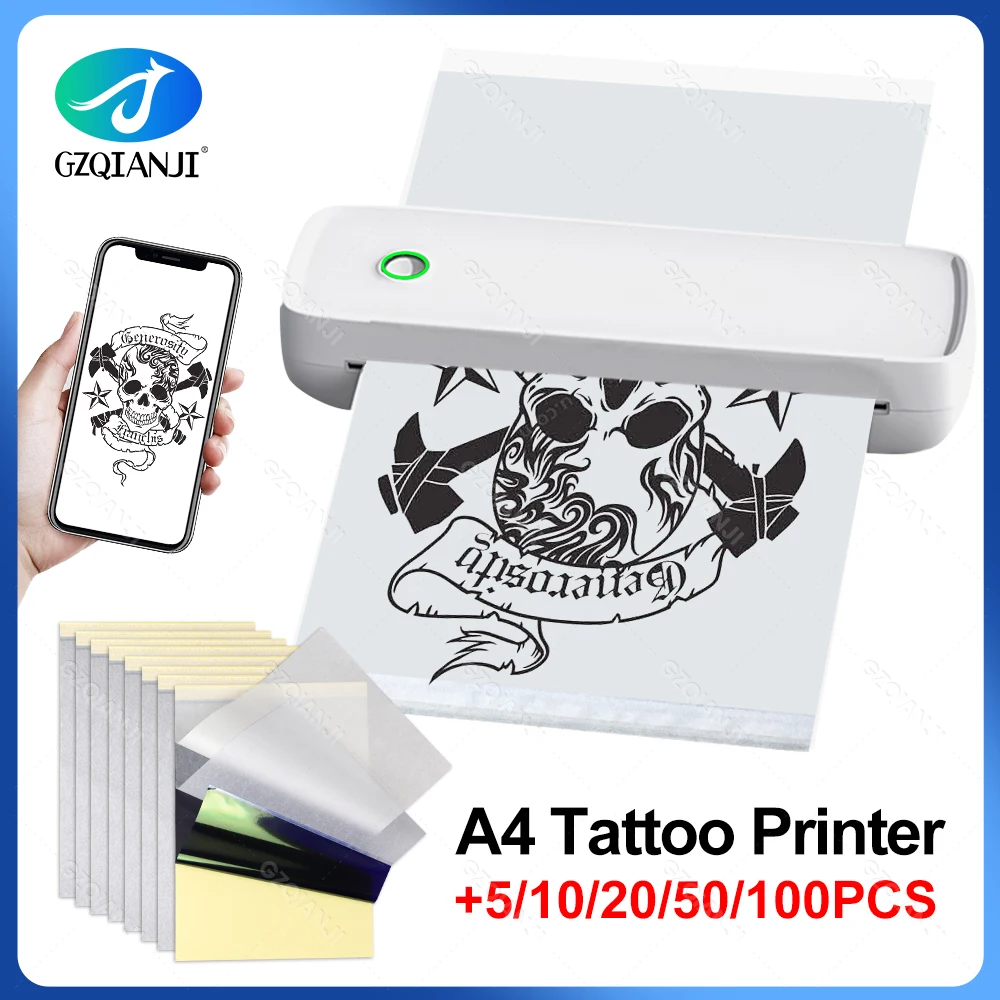The image is an advertisement for an A4 Tattoo Printer by GZQIANJI. The overall design features a blue gradient border that transitions from light blue in the top left corner to dark blue at the sides and back to light blue at the bottom right. In the top left corner, there is a turquoise green to blue gradient oval set against a white background, with "GZQIANJI" written underneath in black text. To the right, there's a depiction of a white printer with an output resembling an upside-down skull with hammers on either side of the head, reminiscent of a skull and crossbones. A Caucasian hand is holding out a cell phone screen, presumably to interact with the tattoo printer. In the bottom right corner, black text reads "A4 Tattoo Printer," with red text below stating "plus 5/10/20/50/100 PCS." Additionally, there are some overlayed images with clear covers to the left side of the advertisement, enhancing the visual appeal and context of the product.